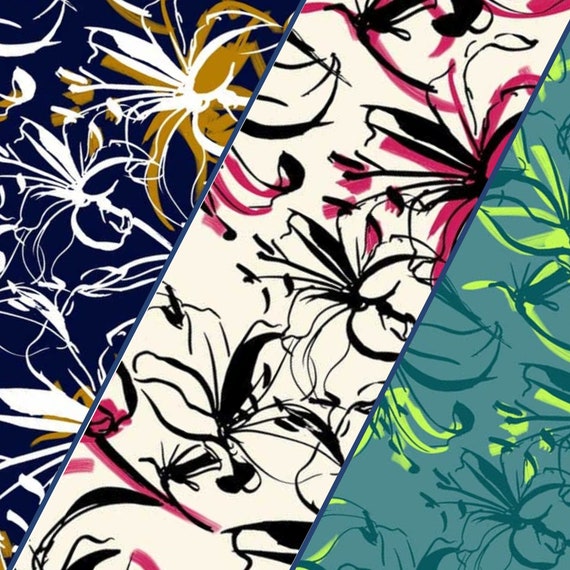The image features a detailed display of three different wallpaper patterns used side-by-side, likely in a room such as Harry's main bathroom. The first wallpaper on the left showcases an aqua background adorned with darker blue flower designs, accented with glow-in-the-dark green details. The middle wallpaper, separated by a distinct blue line, presents white flowers traced in black, set against a beige background with pink highlights. The third wallpaper on the right has a navy background featuring white flowers with brown accents. Together, these diverse and vivid designs create a unique and visually striking arrangement.